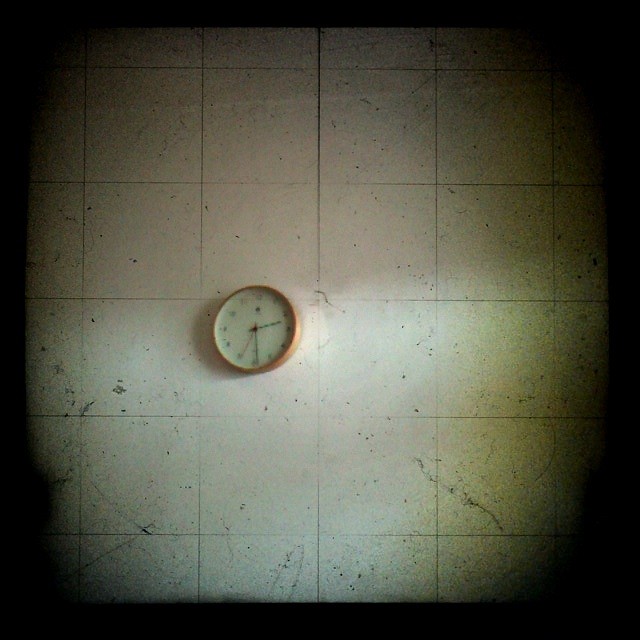This image features a computer-generated rendering or a highly grainy photograph of a wall-mounted clock positioned nearly at the center of the frame. The wall itself is composed of large, square tiles that have a marble-like appearance, characterized by subtle, natural stone-like patterns. The clock seems to blend with these tiles, giving an impression of being carved from marble, and exhibits a slight transparency against the wall.

The clock is circular with a striking orange border that provides a vivid contrast to its surroundings. Its face is off-white, presenting a gentle yet noticeable background for the time indicators. The clock's minute, hour, and second hands are all black, standing out sharply against the lighter clock face. The time displayed is 2:28, with the second hand precisely pointing at 34 seconds.

Despite the graininess, the numbers 1 through 12 are present around the clock face, although they are barely visible and somewhat obscured by the low image quality. Directly beneath the number 12, there is a small black dot on the clock face, adding a unique element to its design. The overall composition of the image captures both the elegance of the marble-like materials and the intricate details of the clock itself.